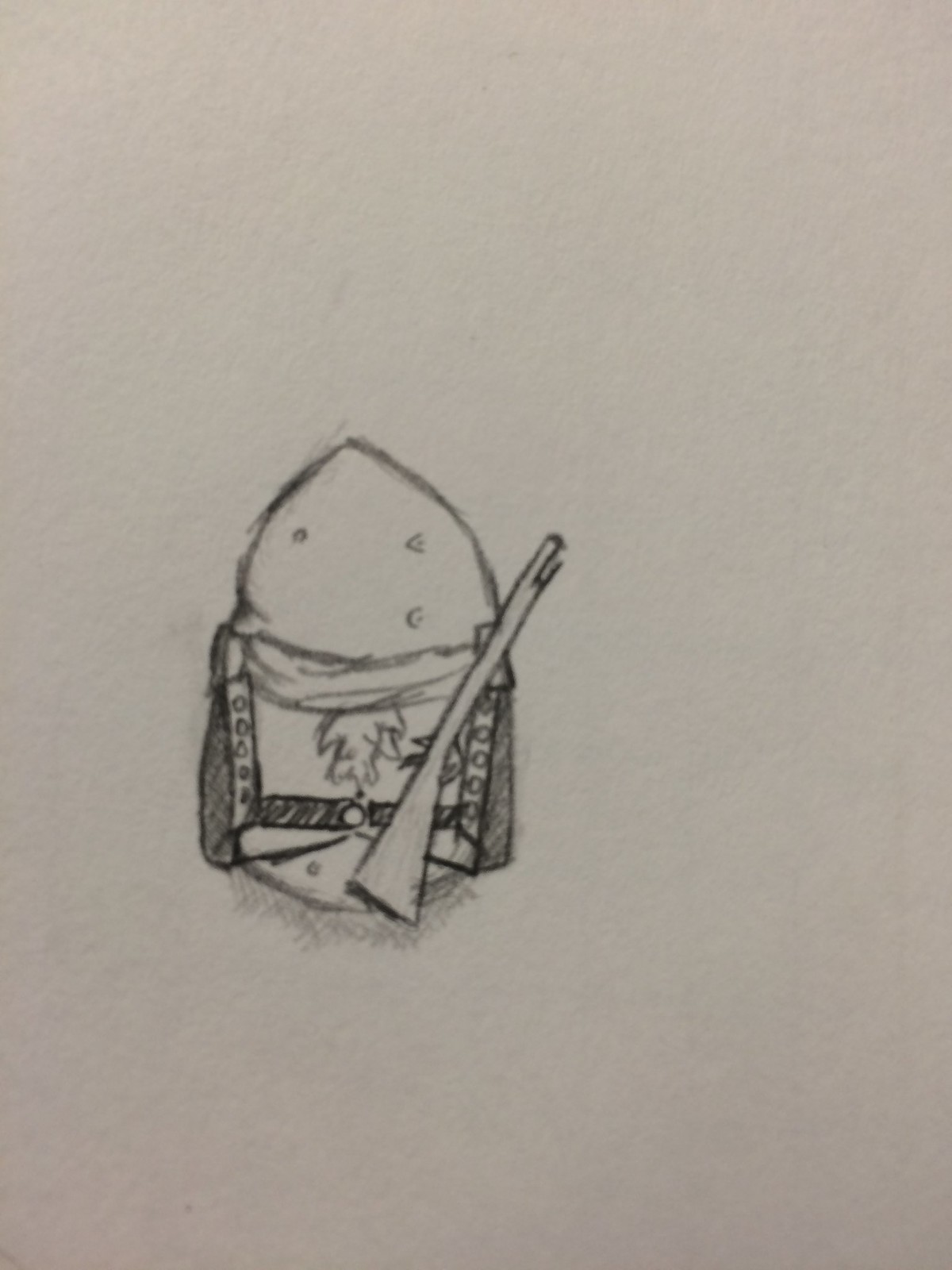A detailed pencil illustration on white paper depicts an anthropomorphic potato character dressed in a detailed uniform. The potato figure is adorned with a comprehensive outfit, including a distinctive scarf and a shirt featuring an emblem that resembles a flame. The shirt's sides are fastened by buttons, and a belt cinches the character's waist. It holds a long rifle with a prominent buttstock pointing to the right. The rifle is meticulously drawn, highlighting its length and structure. A subtle shadow beneath the character adds depth to the image. The potato itself is textured with numerous tiny circles, enhancing its lifelike appearance.